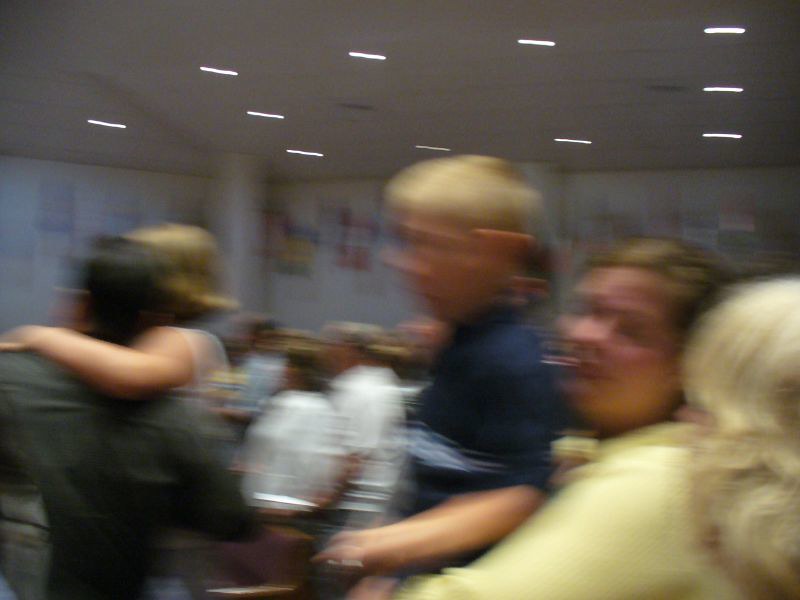This is an indoor photo that appears to have been taken while the camera was in motion, resulting in a heavily blurred image. Multiple light fixtures are visible on the ceiling, illuminating the scene. In the center of the room, a distinctive round metal pole emerges from the floor, surrounded by a group of people. The back wall is adorned with several posters, adding some context to the setting. 

In the foreground, a man wearing a black shirt is holding a little girl, while a woman in a long-sleeved yellow shirt is seen carrying a blonde-headed boy dressed in a navy blue polo shirt with a white stripe. The woman's face is slightly turned toward the camera, though her body faces left. On the bottom right, another figure's blonde hair is faintly visible behind the woman in the yellow shirt. Off to the very far right, a blonde woman with shoulder-length hair can be seen. Most people in the image seem to be facing left and somewhat to the back, with a couple in white shirts positioned centrally but slightly further back.